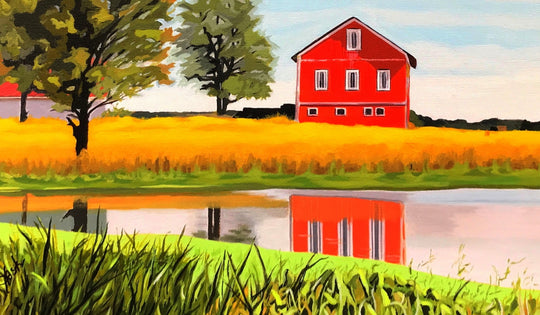This image is a detailed painting executed in a watercolor style, featuring soft brushstrokes. Dominating the scene is a red, three-story barn with a black roof and white trims around its windows. The barn's structure is reflected vividly in the tranquil pond that extends across the middle of the painting. The foreground is characterized by distinct green leaves and shaggier vegetation at the bottom border. Moving further into the painting, the field transitions into an orange-golden hue, suggesting crops like corn or wheat. On the far side of the pond, the landscape is dotted with yellowing tall grass. There are three trees to the left of the barn, painted with splotchy green foliage, and another gray structure with a red roof behind them. The sky above is a clear blue adorned with a scattering of white clouds, enhancing the serene, rural ambiance of the scene.